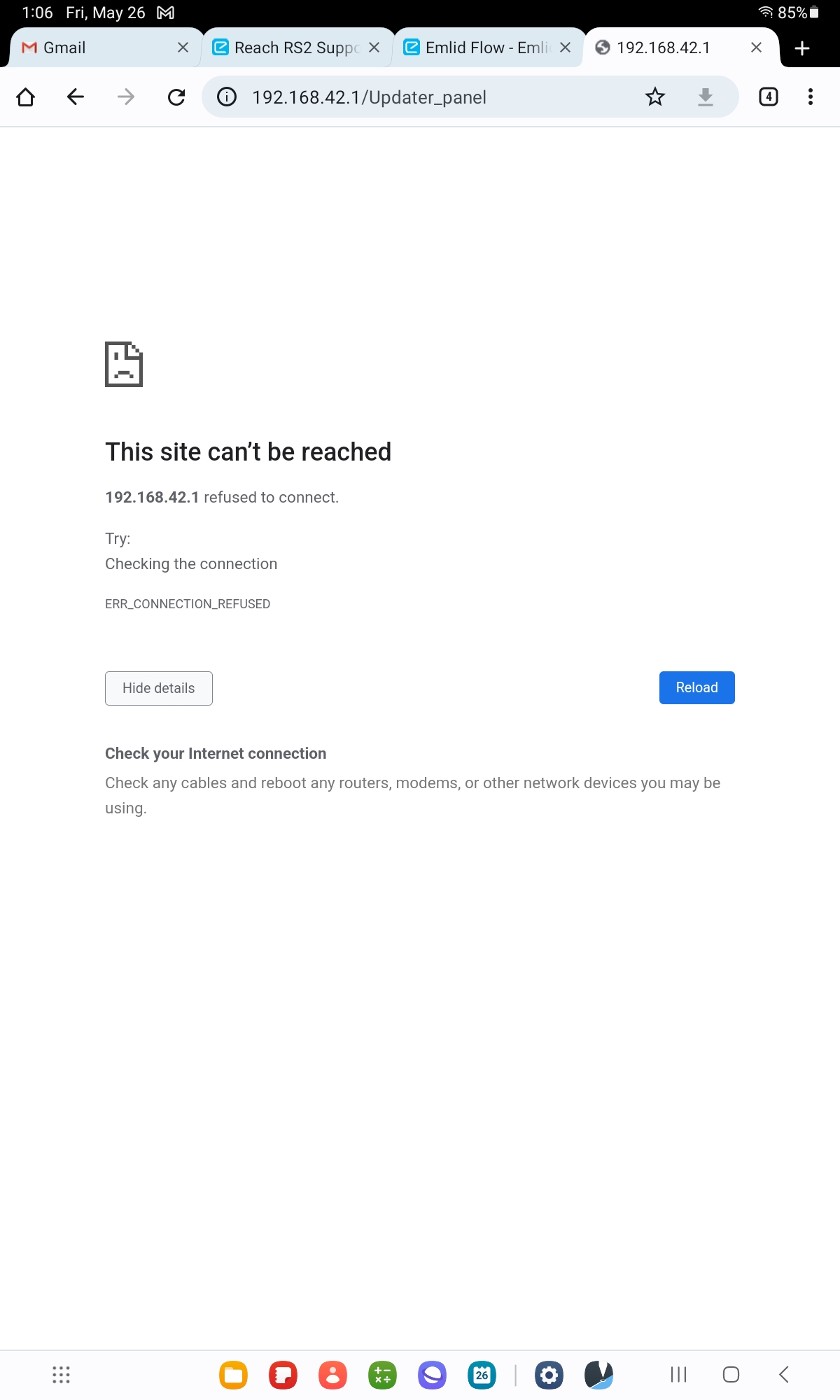A detailed screenshot captures an error page on a tablet device. The screenshot clearly shows the tablet's status bar, where, on the left-hand side, the time "1:06" and the date "Friday, May 26th" are displayed in white font over a black background. On the right side of the status bar, the Wi-Fi icon indicates full signal strength, and the battery icon shows an 85% charge.

The image depicts a browsing session within the Chrome app. Multiple tabs are visible, including ones for Gmail, Reach RS2 support, and Enlid Flow. The active tab's URL is a local IP address: "192.168.42.1". In the address bar, the extended URL reads "192.168.42.1/updater_panel".

The main content of the screenshot is an error message within the Chrome browser that states, "This site can't be reached." Accompanied by a sad-faced page icon, the error message details "192.168.42.1 refused to connect." The error code provided is "ERR_CONNECTION_REFUSED". Below this message are two buttons: a gray "Hide details" button and a blue "Reload" button. Additional troubleshooting guidance at the bottom advises the user to check their internet connection, cables, and to reboot any network devices such as routers or modems.